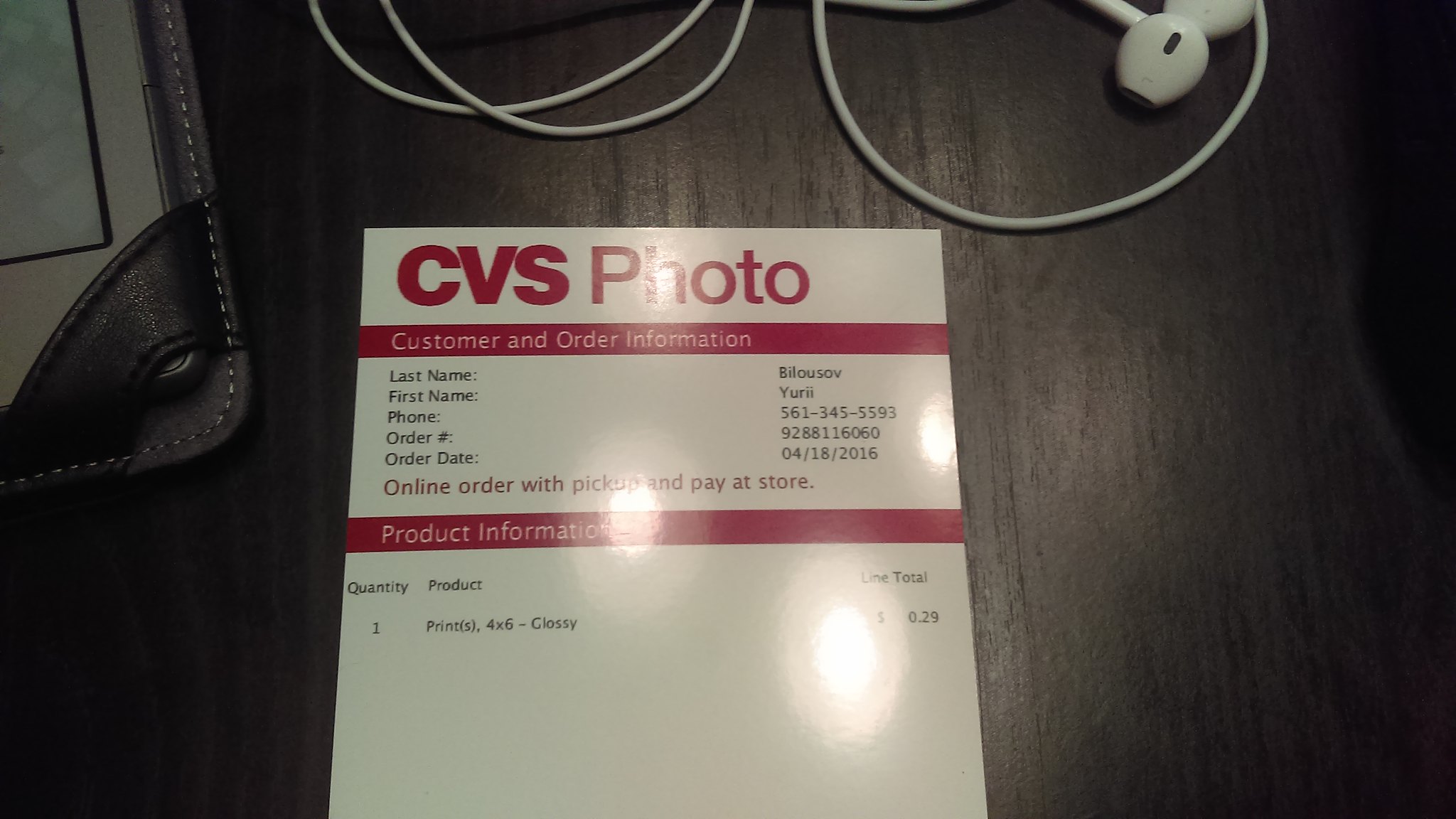The photograph captures a CVS Photo order receipt prominently displayed on a dark-colored wooden desk, likely black or very dark brown. The desk surface reveals a rich wood grain pattern. Positioned above the receipt is a pair of white corded earbuds, possibly Apple-branded, adding a casual clutter to the scene. In the upper left corner of the image, the edge of a dark, likely black, leather case—partially revealing what might be a tablet or a laptop—adds an element of sophistication.

The CVS Photo receipt itself is stark white, featuring the bold "CVS Photo" heading in bright red letters at the top. Directly beneath this red header, a line of red text demarcates the section titled "Customer and Order Information." This section contains the customer's details: first name, last name, phone number, order number, and the order date, listed in black type. The date noted on the receipt is April 18, 2016.

Further down, the text reads "Order online with pickup and pay at store" in red letters, followed by another red banner indicating "Product Information." The specifics of the order are listed here in black font: a quantity of one 4x6 glossy print with an order total of 29 cents. The photograph exudes an organized yet lived-in feel, emphasizing the mundane yet personal nature of the receipt amidst everyday objects.